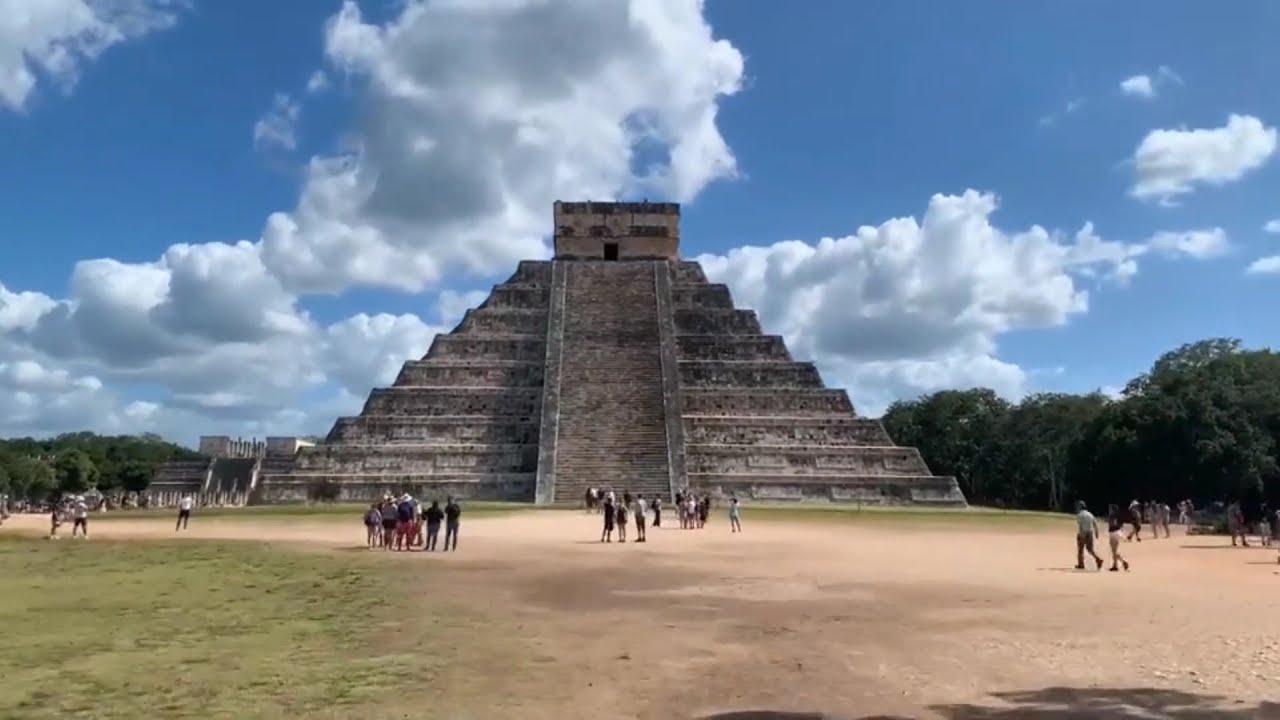The image captures the majestic ancient Mayan pyramid of Chichen Itza in Mexico, prominently positioned in the center with a clear blue sky and wispy cumulus clouds in the background. The pyramid, with its gray stepped structure leading up to a flat top, is characterized by layers that resemble steps ascending to a rectangular summit. Flanking the pyramid are two lines of concrete ramps creating a balanced symmetry. Surrounding the pyramid, numerous individuals are either walking, standing, or gazing at the breathtaking ruin, all dispersed across a sandy, brown, and green terrain. To the left of the pyramid, smaller buildings can be seen, while the background is adorned with lush green trees, adding a natural contrast against the historical stone structure. The open land exudes an inviting daytime ambiance, enriched by vibrant natural light that enhances the color and clarity of the scene.